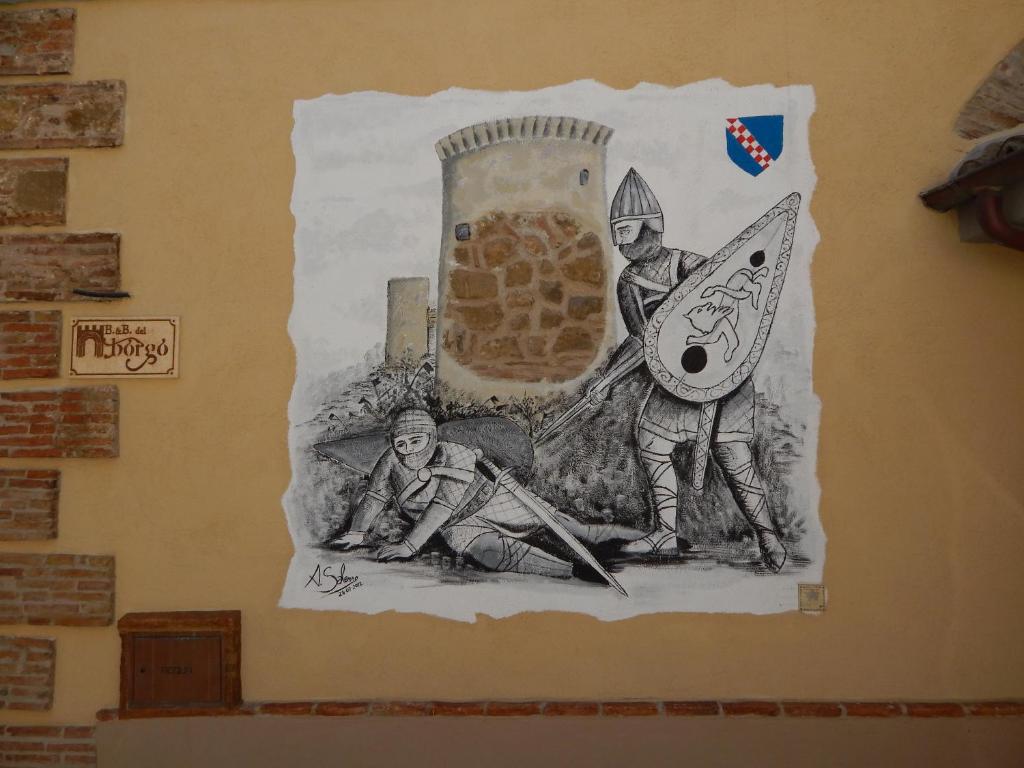The image depicts a detailed painting set against a brown-toned, brick-patterned wall. The bricks, varying from full to three-fourths in visibility, stretch horizontally from the top to the bottom on the left side of the scene. At the very bottom, there is a single row of bricks forming a shelf, on which a small brown box rests. In the middle of the brick wall, a white rectangular plaque with jagged edges showcases a dynamic medieval scene. 

The painting itself features two knights locked in combat. The knight on the right, donned with a pointy metal cone-shaped helm, holds a teardrop-shaped shield emblazoned with a lion and a sword pointed towards his opponent. This knight also wears leather straps on his sandals. Meanwhile, the other knight is on the ground, his hands planted firmly while he looks to his left, his nose and eyes visible while his mouth is covered by a guard. A sword lies beside him as he appears to be attempting to crawl away. The scene is rendered in black and white, giving it a sketched appearance, while a brown tower and a crest of blue with red and white checkered squares embellish the background. The left side of the brick wall features a plaque reading "B&B Del Borgo."